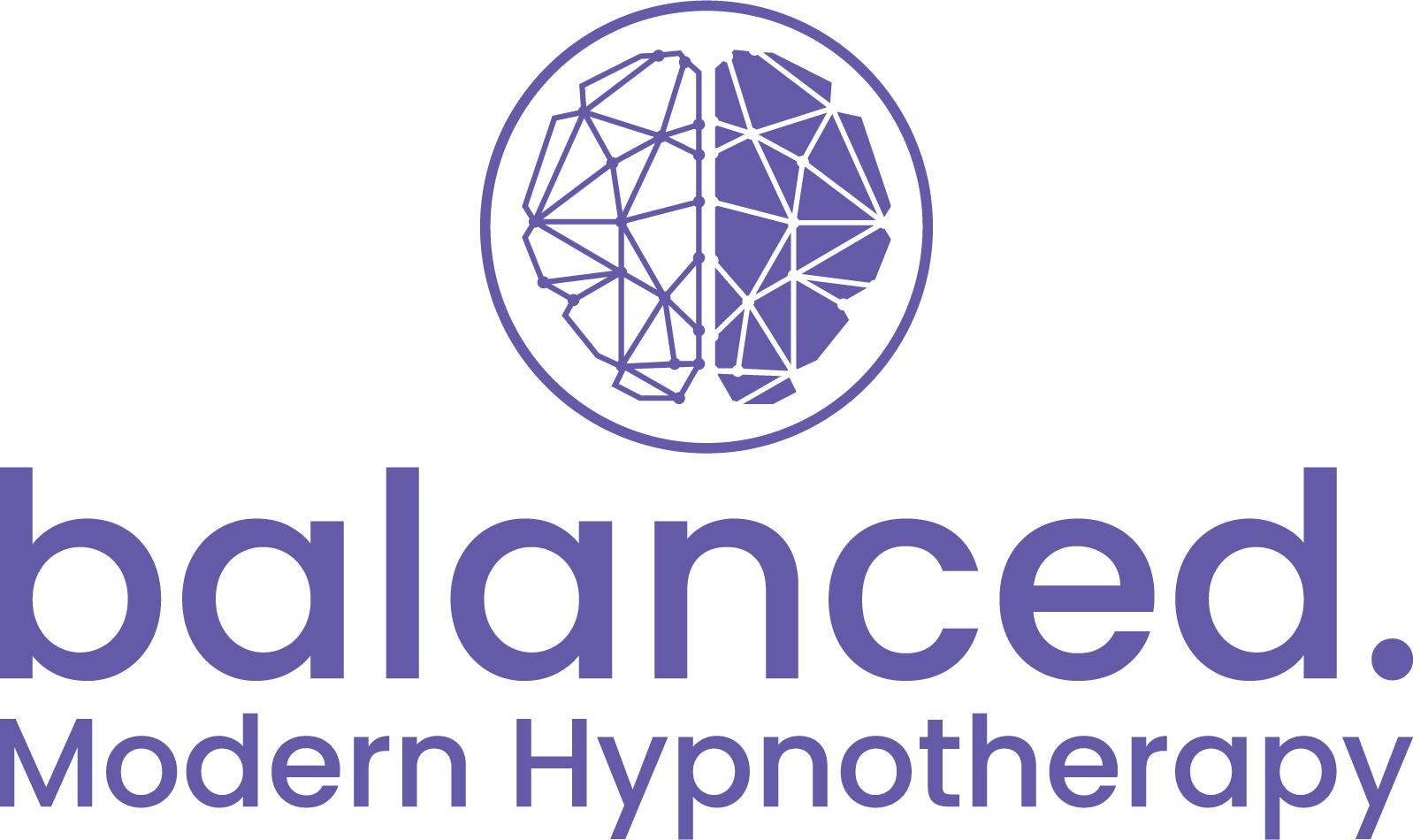The image is a graphic design logo set against a white background in landscape orientation. At the top center of the image is a round circle featuring a stylized illustration of a brain, divided into two hemispheres. The right hemisphere is depicted as a solid purple shape with intricate white lines forming triangular and diamond patterns. The left hemisphere is a white shape adorned with purple lines creating similar geometric patterns. The entire illustration is encircled by a thin purple outline. Below the circle, in bold, elongated, lowercase purple text, the word "balanced." appears. Underneath this, in a smaller font and also in purple, is the phrase "Modern Hypnotherapy," with 'Modern' and 'Hypnotherapy' both capitalized. The composition is clean and emphasizes the modern and balanced theme through its use of color, shape, and typography.